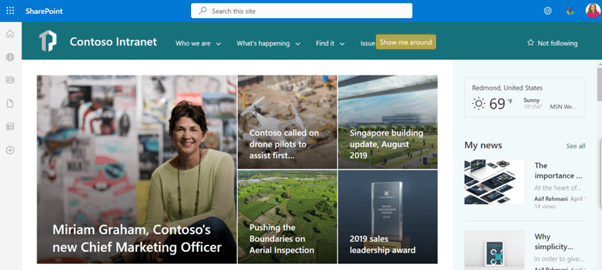Screenshot of a SharePoint webpage displaying the Contoso Intranet. At the top left corner, the title "SharePoint" is prominently displayed within a blue banner with white text. On the right side of the banner, there's an icon of a person's face, along with two other icons. Centrally positioned at the top of the page is a white search bar with a magnifying glass icon.

A teal banner runs below the top section, featuring an icon and the bold text "Contoso Intranet". Adjacent to this are navigation links labeled "Who We Are," "What's Happening," "Find It," "Issue," and a "Not Following" label with a star icon. A rectangular mustard-colored button labeled "Show Me Around" is also visible.

On the left side of the page, a vertical menu displays several icons: a house, a circle, a rectangle, a document, another shape, and a plus sign.

The main content area showcases a large image of a woman, captioned "Miriam Graham, Contoso's new Chief Marketing Officer." Beside this, a smaller square reads "Contoso Calls on Drone Pilots to Assist First." To the right, there's a headline "Singapore Building Update August 2019," followed by another titled "Pushing the Boundaries on Aerial Inspection." Further to the right is the caption "2019 Sales and Leadership Award."